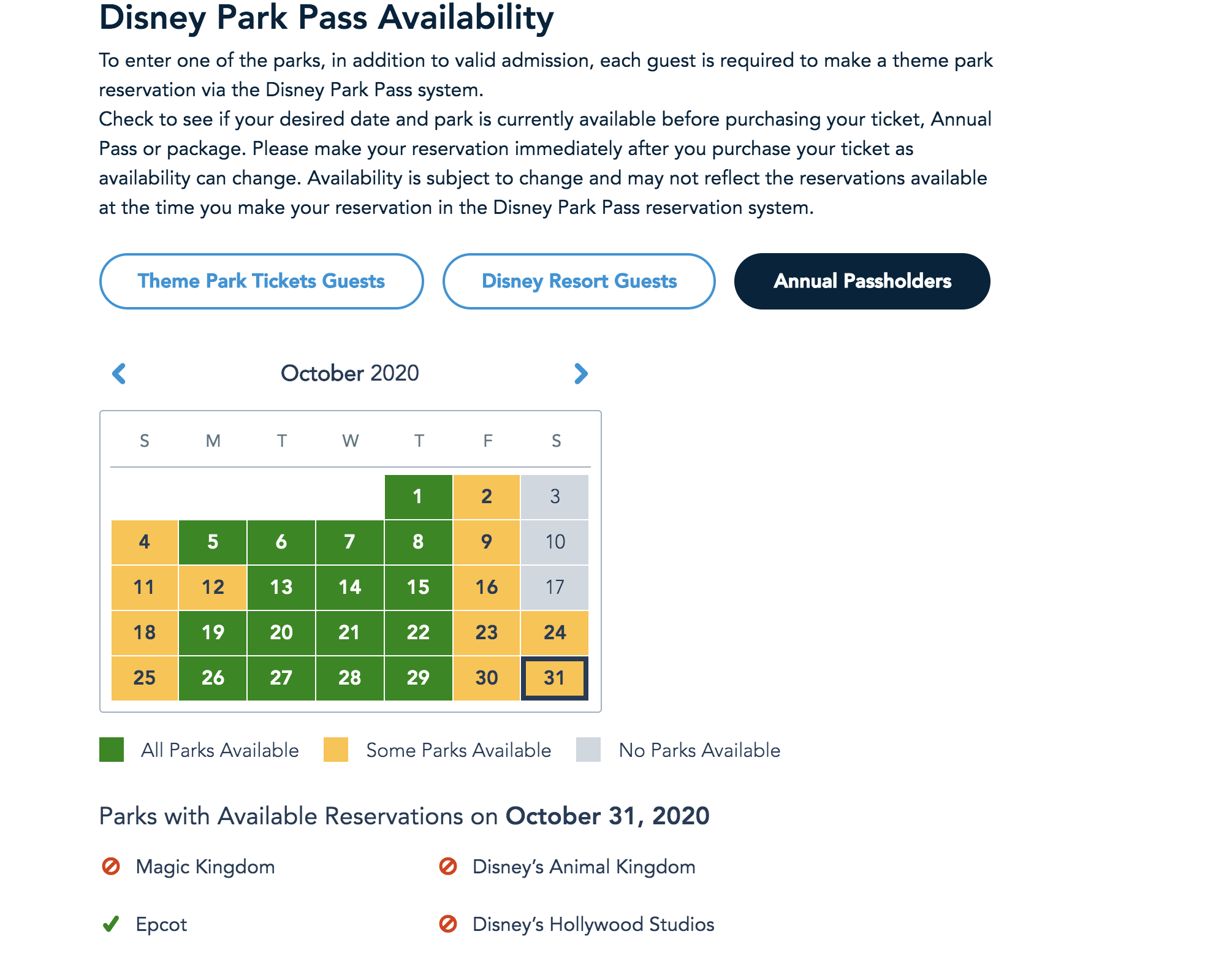This image showcases the Disney Park Pass availability on the official website. The text highlights important information for guests planning to visit Disney parks. It states that in addition to valid admission, each guest must make a theme park reservation via the Disney Park Pass system. Visitors are advised to check the availability of their desired dates and parks before purchasing tickets. It is crucial to make reservations immediately after purchasing tickets, as availability can change.

In the image, there are three distinct categories shown with circular icons: "Theme Park Tickets Guests" in blue, "Disney Resorts Guests," and "Annual Pass Holders," with the latter highlighted in black. The calendar displayed is for October 2020, organized from Sunday to Saturday. The availability status is color-coded: green indicates all parks are available, yellow signifies some parks are available, and gray means no parks are available.

For October 31st, 2020, the chart shows that specific park availability includes:
- Magic Kingdom: Not Available
- Epcot: Available (indicated by a green check)
- Disney's Animal Kingdom: Not Available
- Disney's Hollywood Studios: Not Available

The legend clarifies the color coding used to depict park availability: green (all parks available), yellow (some parks available), and gray (no parks available).